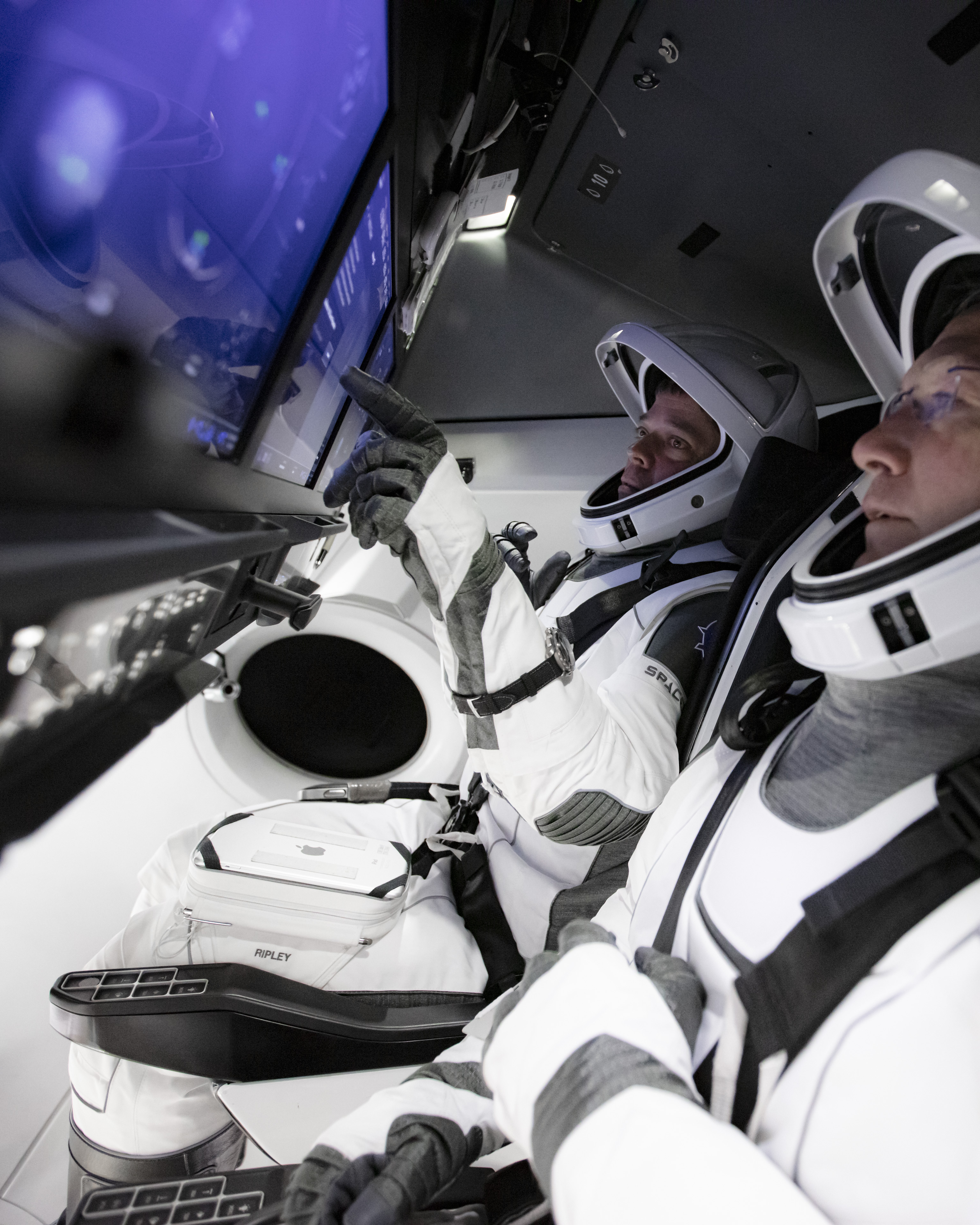Inside the cockpit of a space module, two astronauts are seated side by side, facing left, giving us a side view. They are both dressed in white astronaut suits adorned with black and gray accents. The astronauts' helmets, with raised visors, reveal middle-aged faces, and one of the astronauts wears wired-rimmed glasses. Strapped into their seats with black seatbelts, they sit in front of at least three blue screens displaying white lettering, accompanied by an array of black knobs and control buttons below. The astronaut farthest from the viewer, identifiable by a black-gloved hand, is pointing at the middle screen. Above and to the right, a white light mainly illuminates this astronaut. Both astronauts appear to be intently focused on the screens. Notably, a black patch on the nearer astronaut’s left arm bears the word "Space." The cockpit features gray panel walls, black armrests with additional white buttons, and a white floor, all contributing to the high-tech atmosphere of this space module interior.